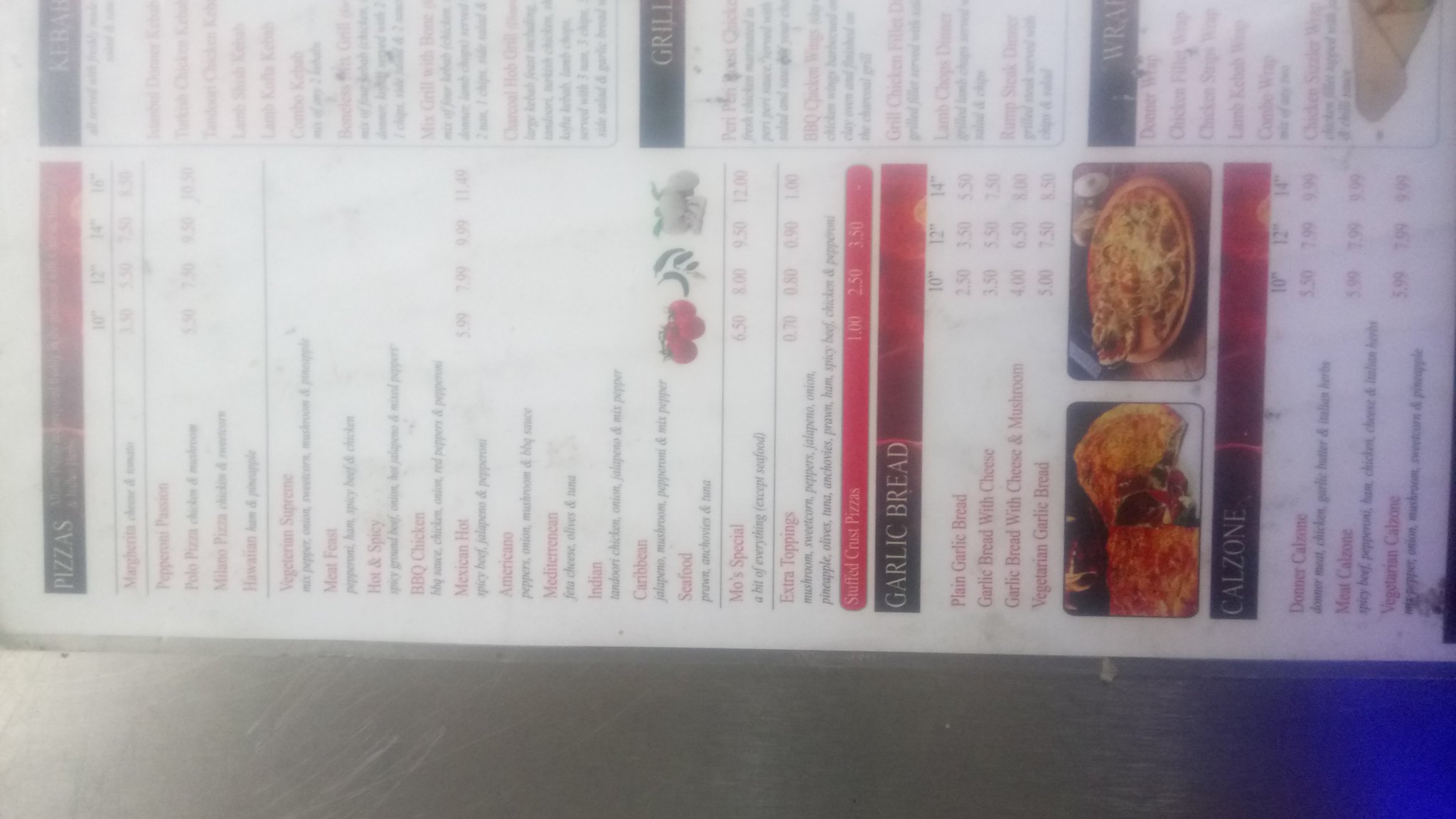This is a photograph of an Italian-themed menu, positioned sideways, requiring viewers to tilt their heads for a proper view. The image captures the menu resting on a steel table, with the surrounding environment suggesting that it was taken at night, given the poor, artificial lighting. 

The menu is arranged in two main columns. The first column, marked by a red banner, lists various pizza options. The pizza names are in red, while their ingredients are detailed in black text. Some clearly visible options include Pepperoni, Pesto, Pasta, Vegetarian, Supreme, and Seafood. Below the pizza section, another red banner highlights extra toppings, followed by a section on garlic bread with several variants like plain garlic bread, garlic bread with cheese, garlic bread with cheese and mushrooms, and vegetarian garlic bread, each offered in sizes of 10, 12, and 14 inches. 

Further down, the menu features images of calzones beneath another red banner labeled "Calzone." The types of calzones listed are Donor Calzone, Meat Calzone, and Vegetarian Calzone. 

The second column starts with a section in a black banner dedicated to kebab options, providing around six or seven choices. Below the kebabs, there's a section for grilled items, although the specific details are illegible. The final part of the menu appears to list various wraps.